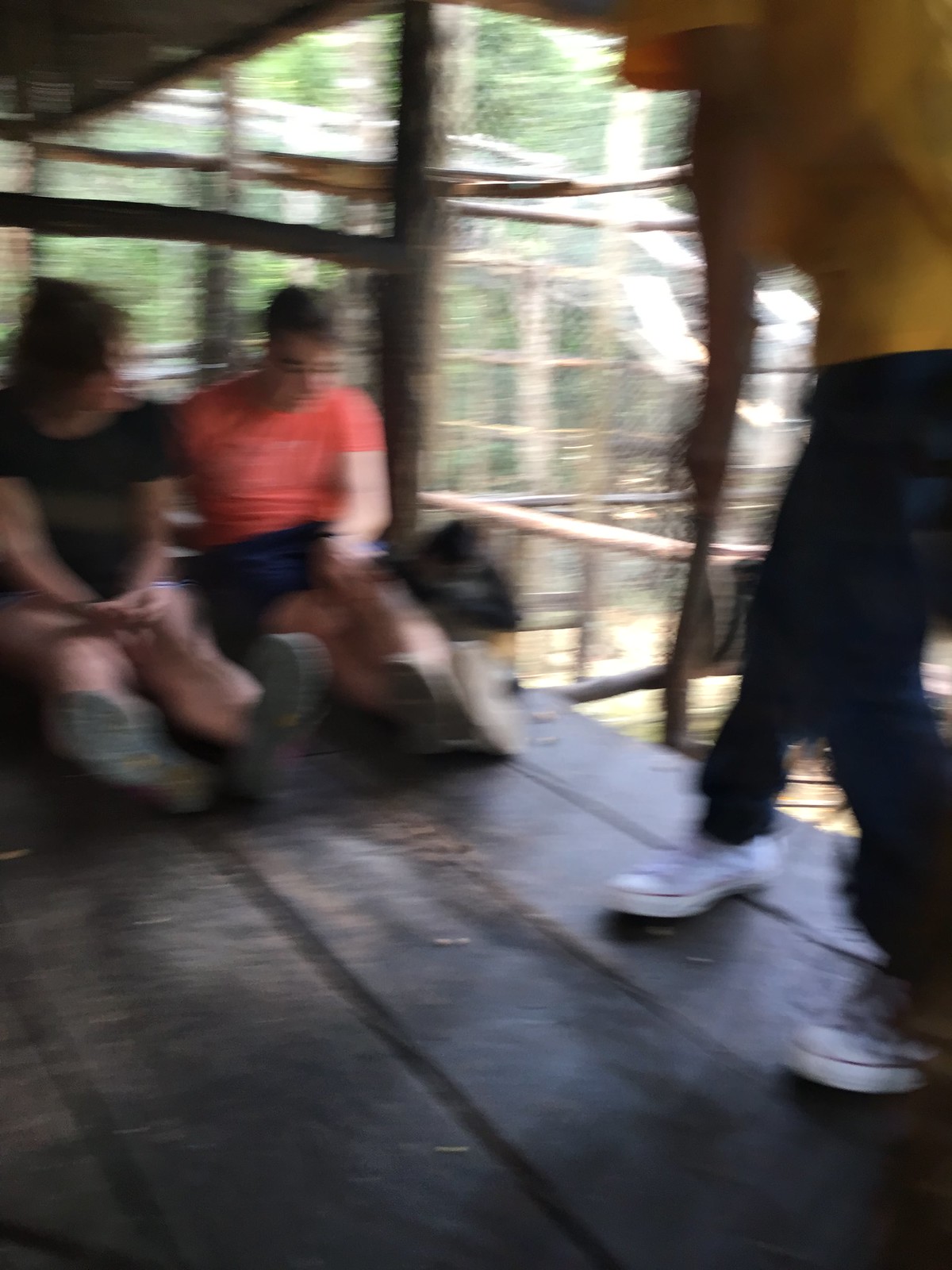The blurred photograph captures three individuals positioned in what appears to be a rustic, elevated wooden structure, possibly a treehouse or an outdoor hut, with thick, uneven planks of black wood that are dirty and dusty. To the far left, a woman with wavy brown hair, wears a short-sleeved black T-shirt, shorts, and hiking or running shoes, while sitting with her legs extended and hands in her lap. She seems to be glancing towards the man next to her. This man, positioned in the center, wears an orange T-shirt, black or blue shorts, and possibly glasses. His legs are crossed, and there is a black bag beside him. To the right of the frame stands a third individual, clad in saggy denim jeans and white Converse shoes. This person, potentially shirtless or wearing a yellow hoodie, is holding something indiscernible due to the blurriness. In the background, there are wooden posts, crossbars, a large chain-link fence, and trees, suggesting an outdoor, nature-bound setting, possibly near animal cages or an aviary, adding to the rugged ambiance of the scene. The image's first-person POV style suggests it was taken in motion.